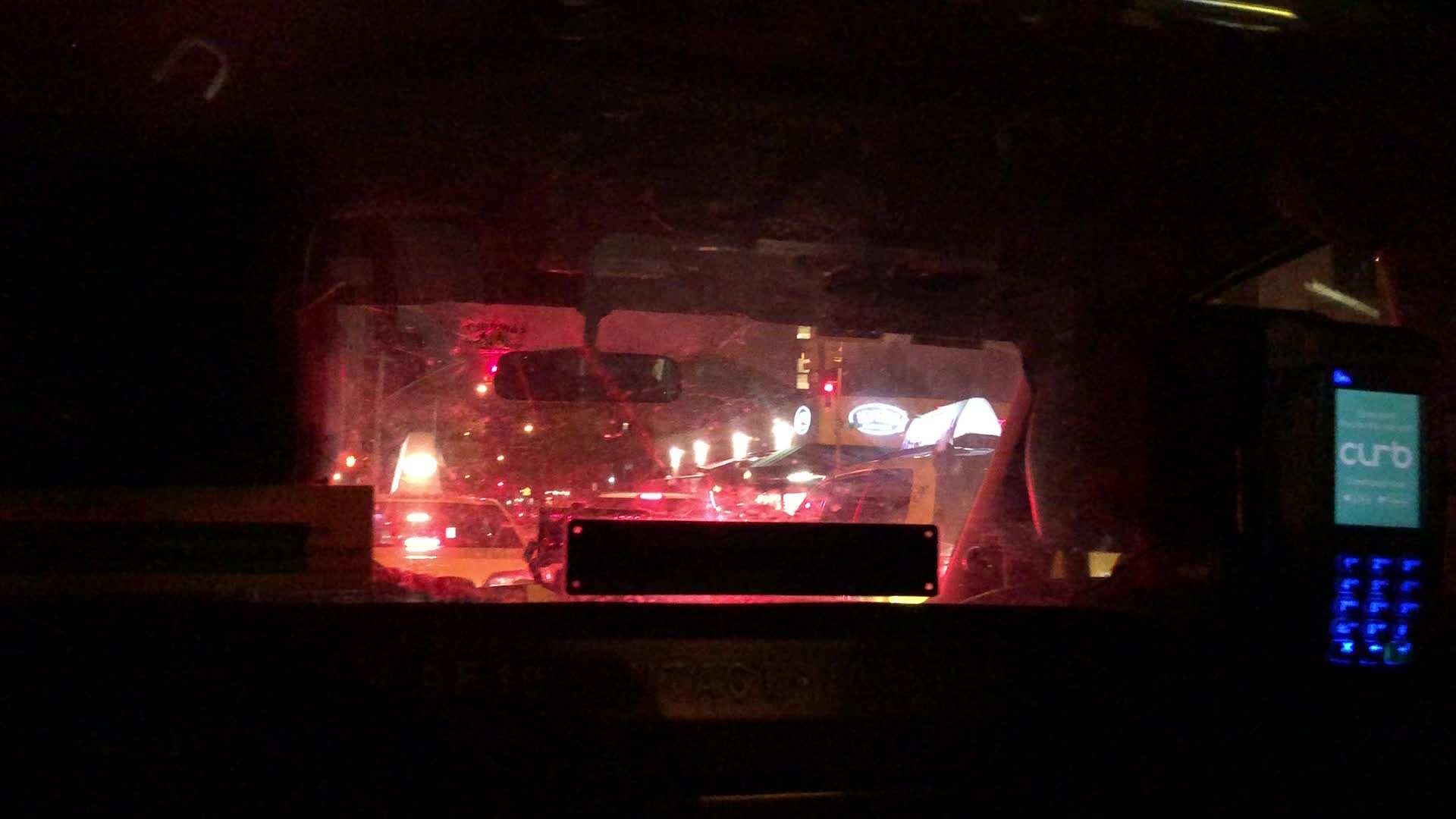This nighttime photograph features a dark background with various illuminated elements. Two cars with lit taxi signs are prominently visible, traveling in opposite directions. On the right side, a row of businesses display vibrant neon signs close to the roofline, adding a colorful glow to the scene. A red traffic light is also visible, contributing to the overall reddish tint that suffuses the image, possibly due to the interplay of the traffic light and other artificial lighting sources.